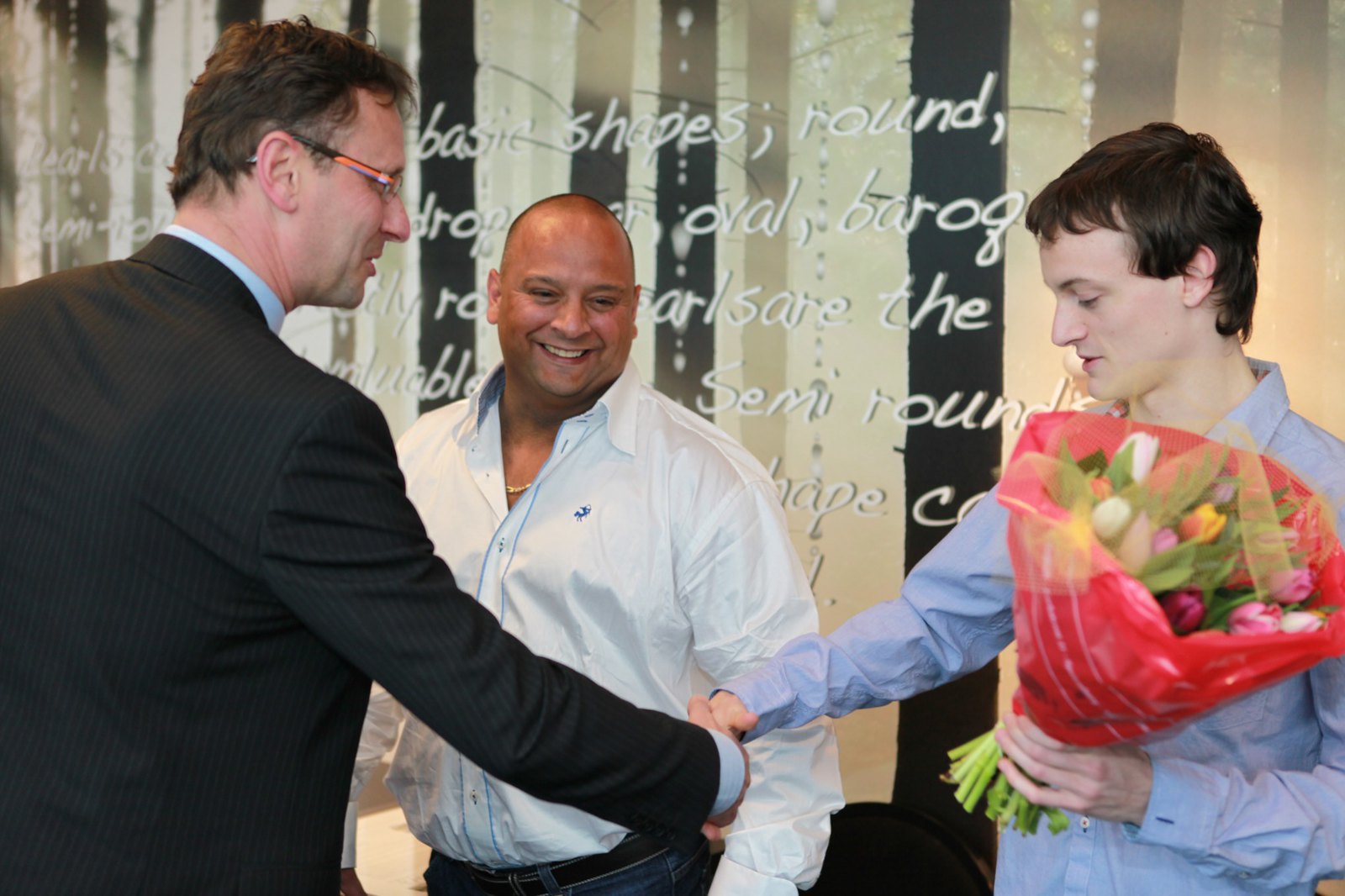The image depicts three men, the central figure being a bald man with a light blue dress shirt, smiling and observing the interaction between the other two men. To his left, a man in his 40s or 50s, clad in a black pinstripe suit with glasses and a light blue dress shirt, is shaking hands with a younger man on the right. The younger man, appearing to be in his late teens or early 20s, is also wearing a light blue dress shirt and is holding a bouquet of flowers wrapped in red cellophane, comprising white, yellow, and pink tulips, with green stems visible at the bottom. The background features drapes with printed statements such as "basic shapes: round, oval, baroque, semi-round." The setting is primarily dominated by colors white, black, blue, red, yellow, and pink. The younger man looks down shyly, while the older man in the suit seems to be speaking to him during the handshake.